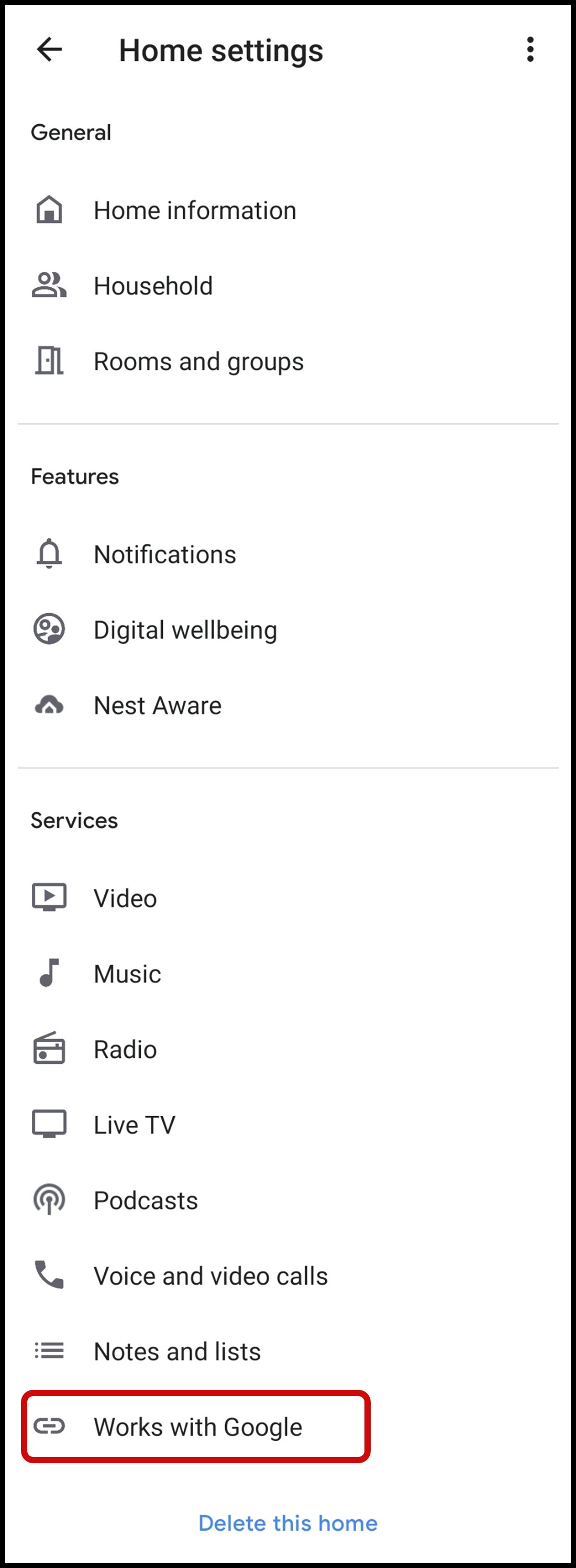The image displays a detailed screenshot of a settings panel, which is a tall rectangular interface predominantly white in background with black text. At the top left corner of the panel, there's a left arrow pointing back, followed by the title "Home Settings" to its right, and three vertical dots at the very far right, likely indicating a menu.

The panel contains three main sections, each with its own title and subsections:

1. **General**:
   - Home Information
   - Household
   - Rooms and Groups

2. **Features**:
   - Notifications
   - Digital Wellbeing
   - Nest Aware

3. **Services**:
   - Video
   - Music
   - Radio
   - Live TV
   - Podcasts
   - Voice and Video Calls
   - Notes and Lists
   - Works with Google (outlined in a red rectangle)

At the bottom of the panel, there's an option in small blue letters that reads "Delete this Home", indicating an action to remove the current home settings. This rectangular option has a thin black outline around it, making it distinct.

This panel is likely a part of a mobile or computer application designed for managing home settings, allowing users to configure various devices and services within their home environment.